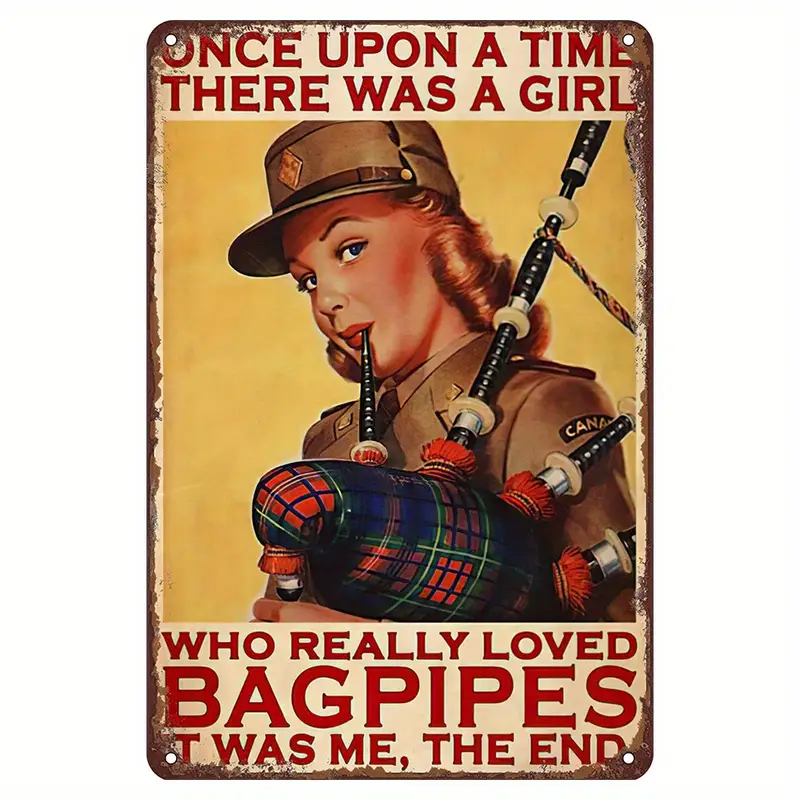This is a detailed color photograph designed as an aged decorative metal tin sign, head-on and weathered at the corners. The sign features a tan background with text at the top and bottom in red font saying, "Once upon a time there was a girl who really loved bagpipes. It was me, the end." The central image is of a young woman in mid-20th-century military uniform with a green hat and matching green attire, adorned with several medals and a visible tie designated for a lady. She has curly blonde hair, striking blue eyes, and bright red lipstick. The woman is playing a Scottish tartan bagpipe with a pattern of blue, green, and red, pressing one pipe to her mouth as if ready to blow. Only visible from the waist up, she gazes directly at the viewer. The sign, which appears to be from Canada, shows pre-drilled holes at the upper corners and evidence of additional nail holes at the bottom, suggesting it has been previously displayed and well-worn over time.